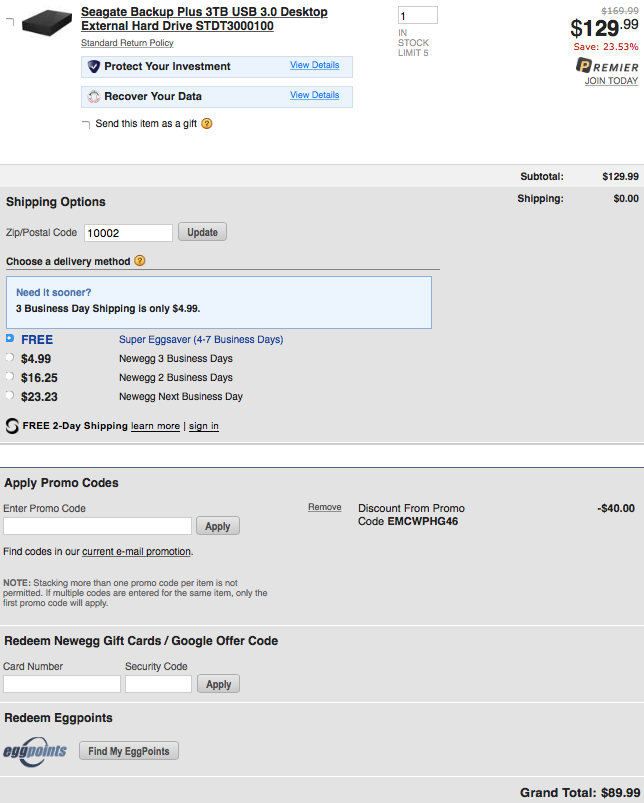Screenshot of an online shopping selection detail page showing a customer’s order. The primary item is a "Seagate Backup Plus 3TB USB 3.0 Desktop External Hard Drive (Model: STDT3000100)." The product, a compact black rectangular box, retails for $169.99 but is currently discounted to $129.99, saving the customer 23.53%.

Key information includes:
- Standard return policy applies.
- Options for protecting the investment and data recovery services.
- The ability to send the item as a gift.
- Quantity selected: 1, with a purchase limit of 5 units.

Highlighted shipping options:
- User's postal code: 10002.
- Various delivery methods ranging from free (4-7 business days) to next business day shipping at $23.23.

Order summary:
- Subtotal: $129.99.
- Shipping cost: Free for 2-day shipping after signing in and learning more about the promotion.
- Opportunity to apply promo codes, with one active code "EMCWPHG46" deducting $40.
- Note on promo code stacking restrictions.
- Options for redeeming gift cards and egg points.

Grand total for the order: $89.99.